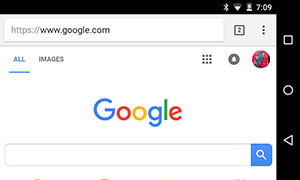The image appears to be a cropped screenshot taken from a mobile phone. On the right side of the black boundary, several icons are visible, including the Bluetooth icon, a half-filled Wi-Fi signal icon, and another small, indiscernible icon, alongside a timestamp displaying 7:09. Below these icons, there is a line of navigation controls represented by a triangle, a circle, and a square.

The screenshot predominantly displays a Google search webpage. At the top of the screenshot, within the search bar, the URL "http://" is shown in gray text, while "www.google.com" stands out in black. Adjacent to the search bar, there is an icon featuring a square with the number two inside it, followed by a set of three vertical dots indicating more options.

Beneath the search bar, the "All" tab is selected, while the "Images" tab is present but inactive. Additionally, there is a grid icon composed of nine dots, a gray circle with a white bell icon representing notifications, and a profile picture placeholder. The iconic multicolored Google logo is centered below these elements. Beneath the logo, a search bar is prominently displayed, featuring a blue button with a white magnifying glass icon on the right side, symbolizing the search function.